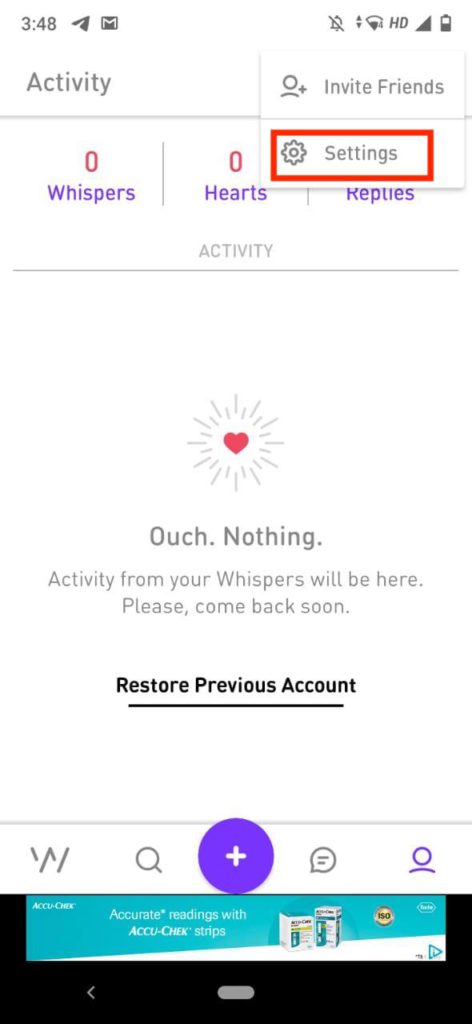The image features a user interface with a clean white background, boasting a resolution of 348 HD. The interface includes options to “Invite Friends” and “Settings,” with the “Settings” button highlighted by a red rectangle. There are indicators for "Whispers" set at zero, "Hearts" set at zero, and "Applause." It displays a message stating, "Activity from your whispers will be here. Please come back soon" and an option to “Restore Previous Account.”

In the interface, various icons are present: a 'W', a magnifying glass symbol for search, a chat symbol, and a profile picture. There's also a blue circle with a white plus sign inside it, indicating an action like adding or creating new content. 

The image also includes two boxes of Accu-Check strips (spelled as "ACCU-CHEK"), though the text is slightly small. At the bottom of the phone screen, there is a black area featuring a less-than symbol (<) and a gray bar.